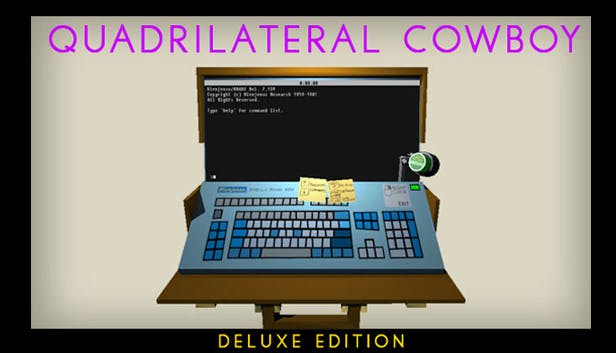The drawing depicts a detailed image of a laptop computer meticulously framed by a black border. At the very top of the image, the title "Quadrilateral Cowboy" is prominently displayed in uppercase purple letters. The laptop itself is set on a brown wooden case, complete with a handle, adding a rustic touch. The keyboard of the laptop is predominantly blue, featuring an array of keys in various shades of blue, gray, and light blue. Slightly above the keyboard, a couple of sticky notes are attached, while the screen displays illegible text against its dark background. At the bottom of the image, "Deluxe Edition" is clearly inscribed in yellow letters, standing out against the neutral background and framed by the surrounding black border.